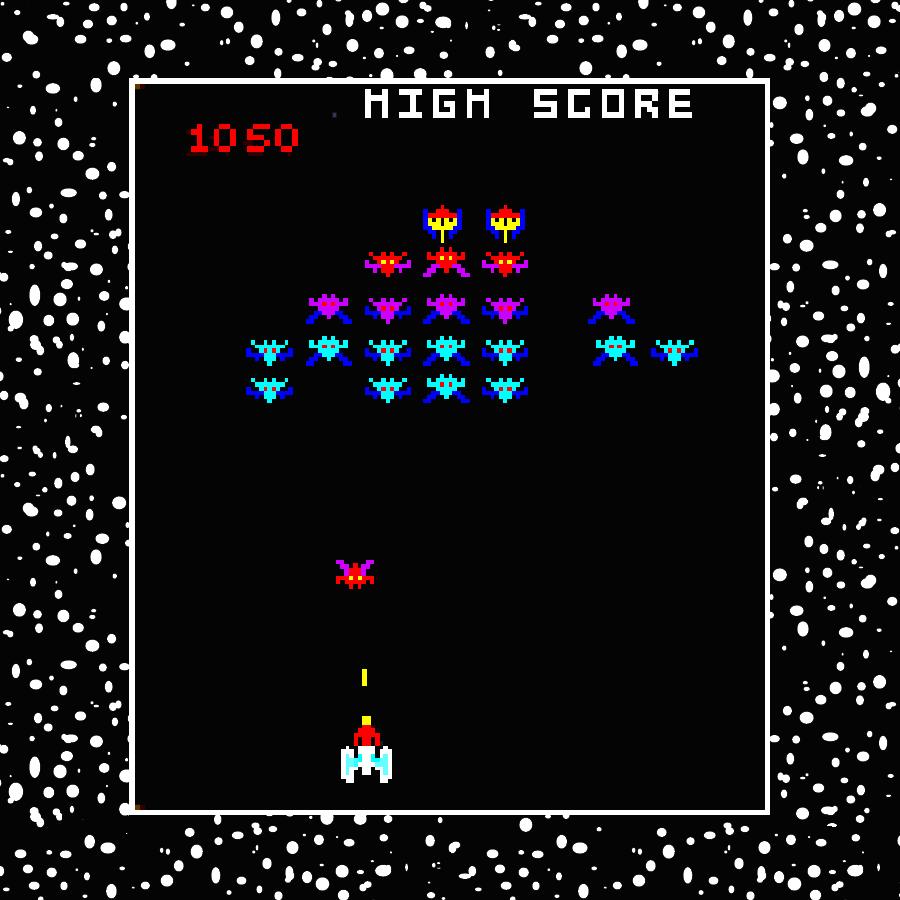This is a screenshot of a classic arcade game, likely from the late 70s or early 80s, featuring very pixelated graphics characteristic of the era. The game appears to be "Space Invaders," displaying a simplistic yet iconic design. The scene showcases a small, pixelated spaceship at the bottom of the screen, actively shooting lasers at rows of alien ships above it. These alien ships are organized in a grid formation with varied colors: teal aliens in the front, purple ones behind them, and gold ones in the back. The background is black with white splotches resembling stars. One alien ship is descending towards the player's spaceship, evoking the tension of the gameplay where the defender must shoot to destroy the invaders. Additionally, a high score of 1,050 is prominently displayed, indicating the challenge and achievement within the game.